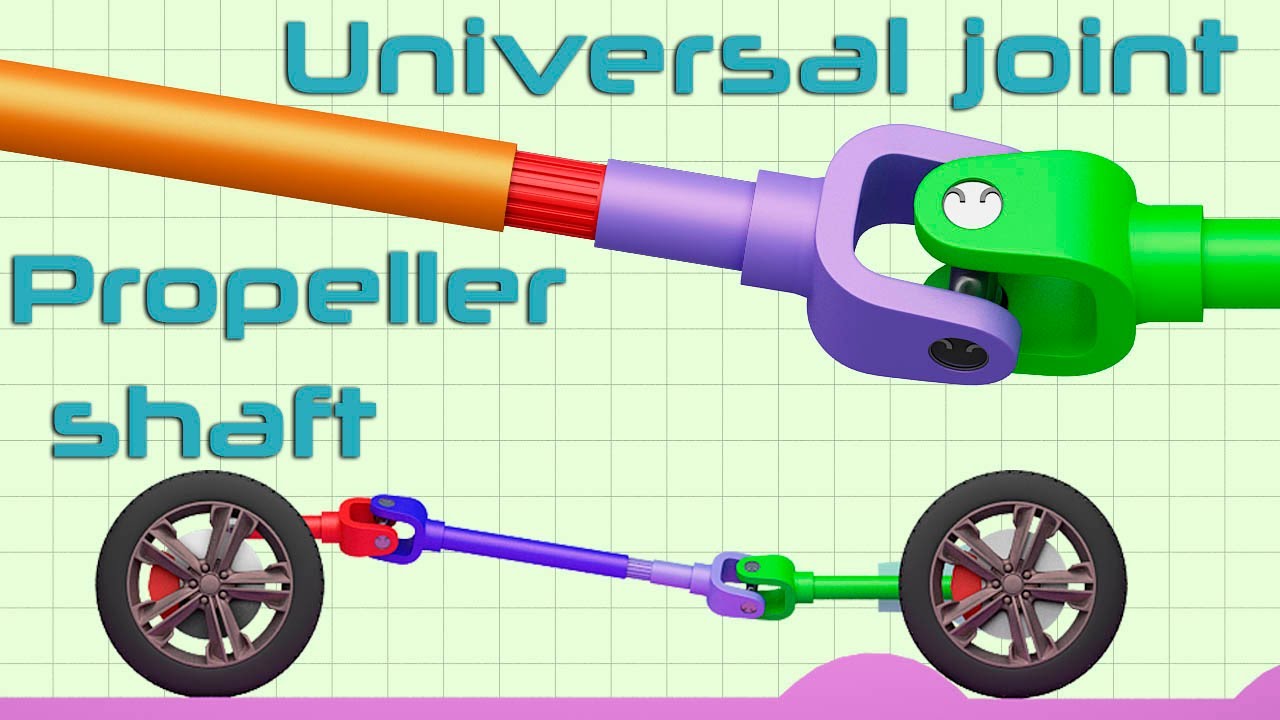This detailed digital illustration, designed to resemble a 3D model, features a labeled depiction of a universal joint. The background mimics graph paper with a series of light blue squares. At the top of the image, bold blue block letters read "Universal Joint," and on the left side, similar blue block letters read "Propeller Shaft." The joint itself is divided into various colored sections, including orange, red, purple, and green, each representing a different part of the joint. The interconnected devices give the impression of two LEGO people holding hands. Beneath the joint, two wheels, resembling car tires, are connected by this multicolored joint structure. The bottom of the image is highlighted by a pink stripe along with a lavender border, adding to its clear schematic presentation.